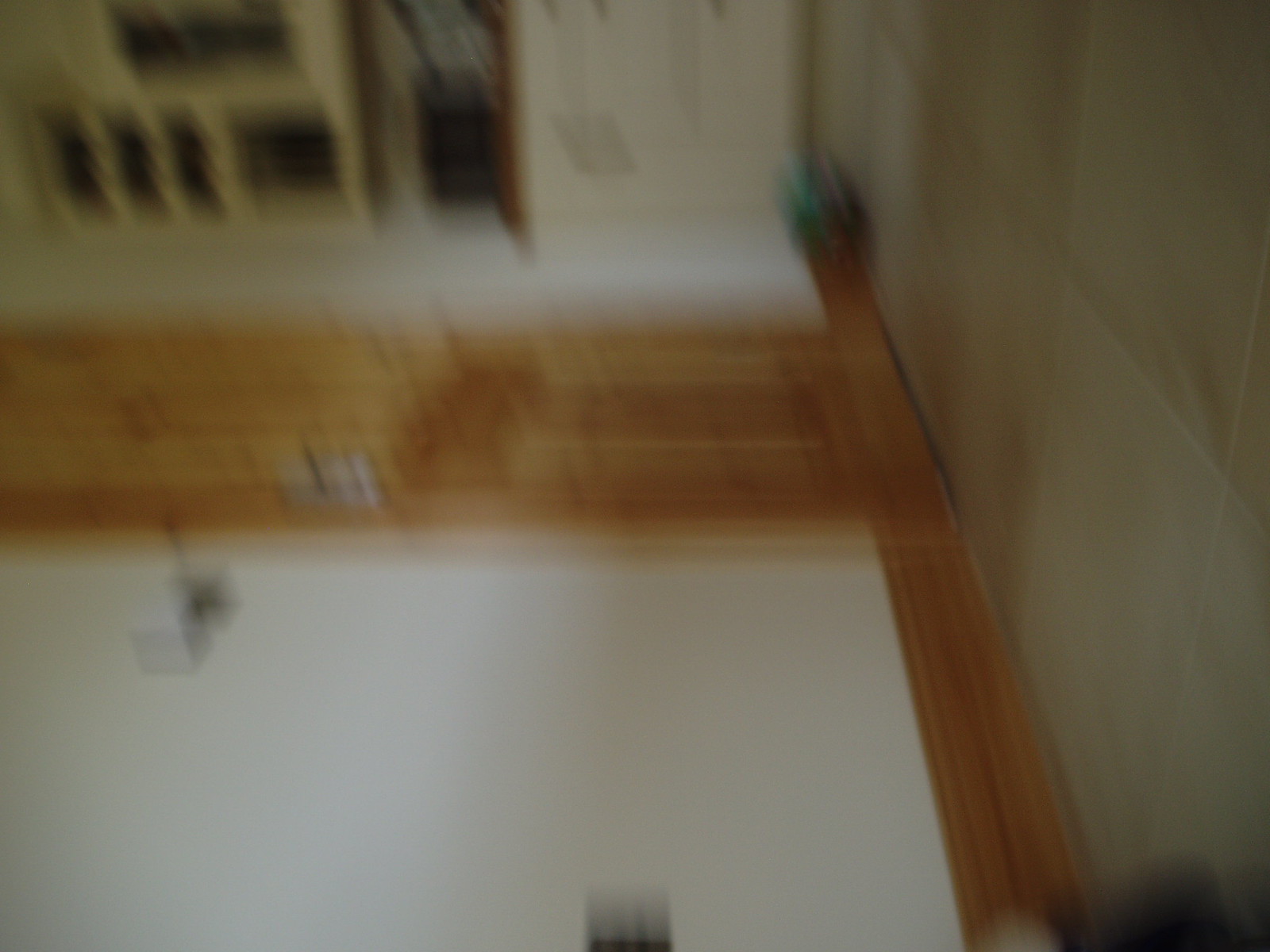This image is notably out of focus and appears to be taken with a rotated camera. Dominating the right side of the photo is a section of stone tile flooring, while the top portion captures white walls. In the center of this composition stands a brown door, characterized by a series of square panels. The middle section of the door seems to be darker, possibly featuring a dark board. Below, the image shows additional white wall space and a brown wooden trim lining. At the very top of the trim, there is a dark object, though its exact nature is indiscernible. In the upper left corner of the image, there are frames mounted on the wall, likely containing photos or artwork.